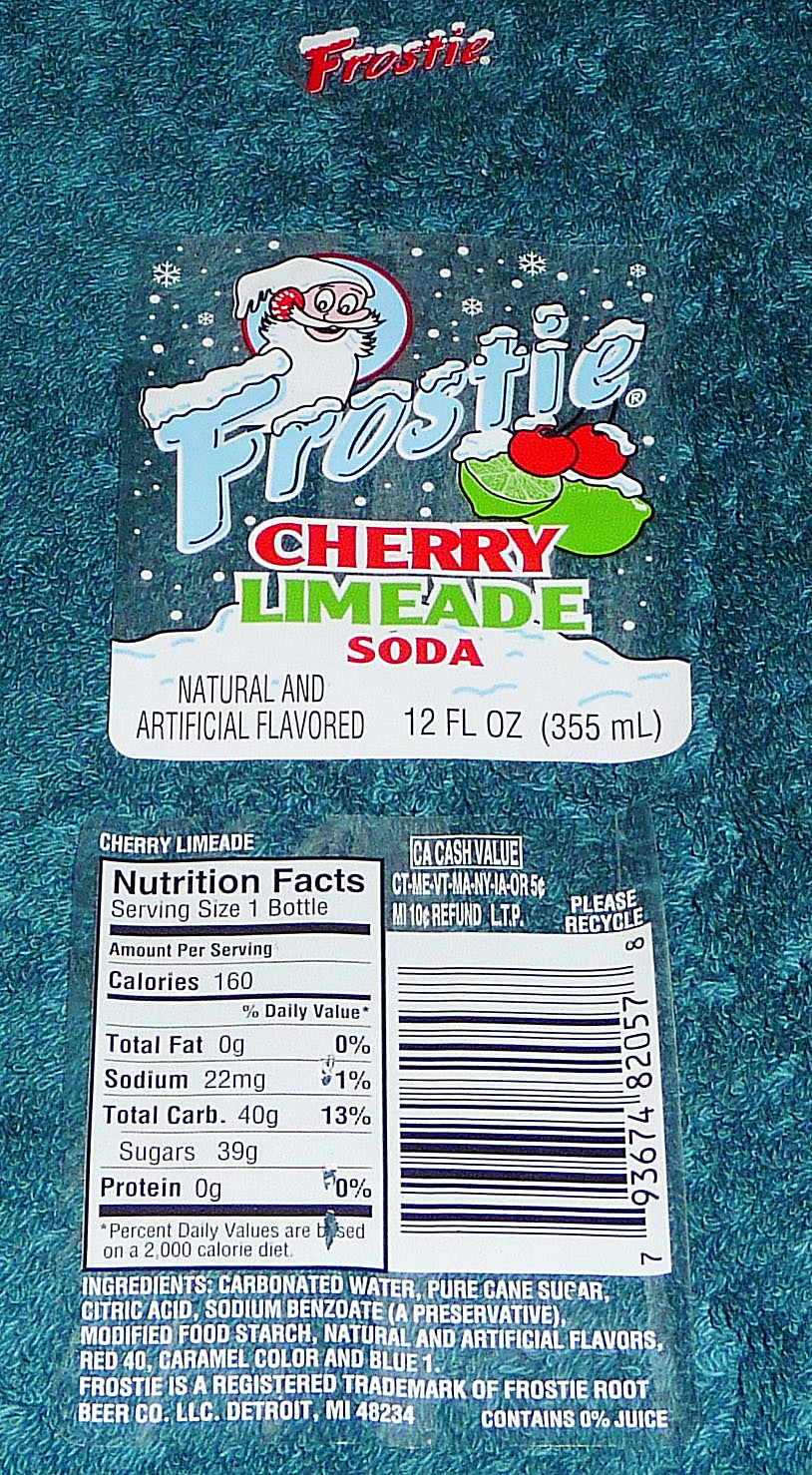The image appears to be of a food product package, specifically a soda can. The prominent feature on the can is the word 'Frosty' written in white or light blue text. Below 'Frosty,' the product is identified as 'Cherry Limeade Soda.' The words 'cherry' and 'soda' are in red text, while 'limeade' is written in green.

Above the text is an illustration of a character with a white beard and mustache, wearing a white hat and a red garment. Adjacent to this illustration are images of cherries and a lime, enhancing the cherry limeade theme.

Underneath the flavor description, it states 'Natural & Artificial Flavor' and '12 FL OZ (355 mL).' Below this information are the nutrition facts: 160 calories, 0 grams of fat, 22 milligrams of sodium, 40 grams of carbohydrates, and 39 grams of sugar. There is also a scannable label on the right side of the package for additional information.

At the bottom of the label, a list of ingredients is provided. All of this is set against a bluish background with an intriguing, slightly hairy texture that adds depth to the design.